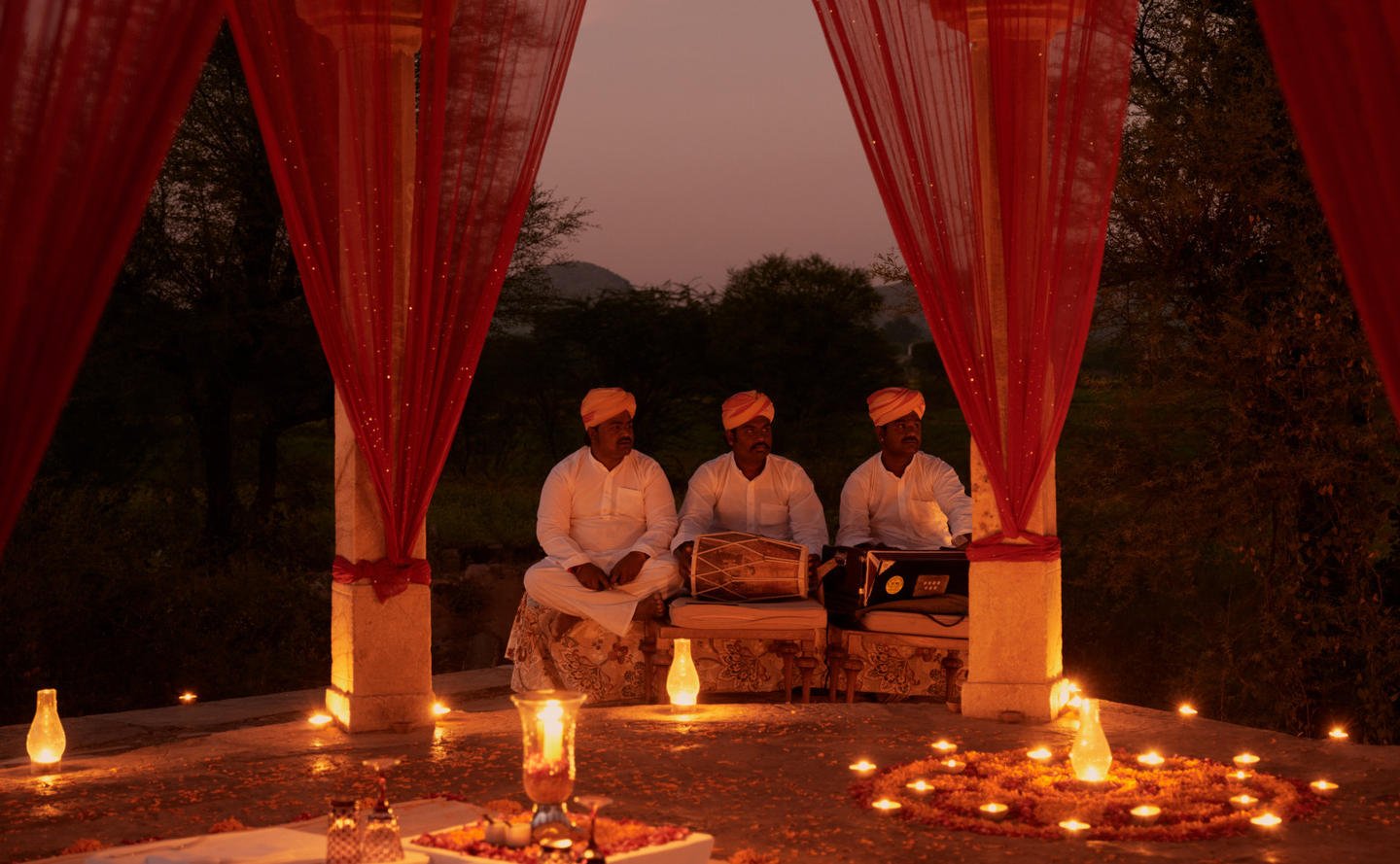Three men, adorned in orange turbans and traditional white outfits, are seated cross-legged on a bench at a ceremonious event. The central figure gently positions a drum in front of him, poised as if ready to play. Candles of varying heights are scattered throughout the scene, casting a warm, flickering glow. Ornate curtains flank the archways surrounding them, with numerous candles nestled within these arches, enhancing the ethereal ambiance. Beyond the archways, the inky night sky forms a backdrop, dotted with dark silhouettes of trees. The men gaze thoughtfully to their left, immersed in the solemnity of the moment.